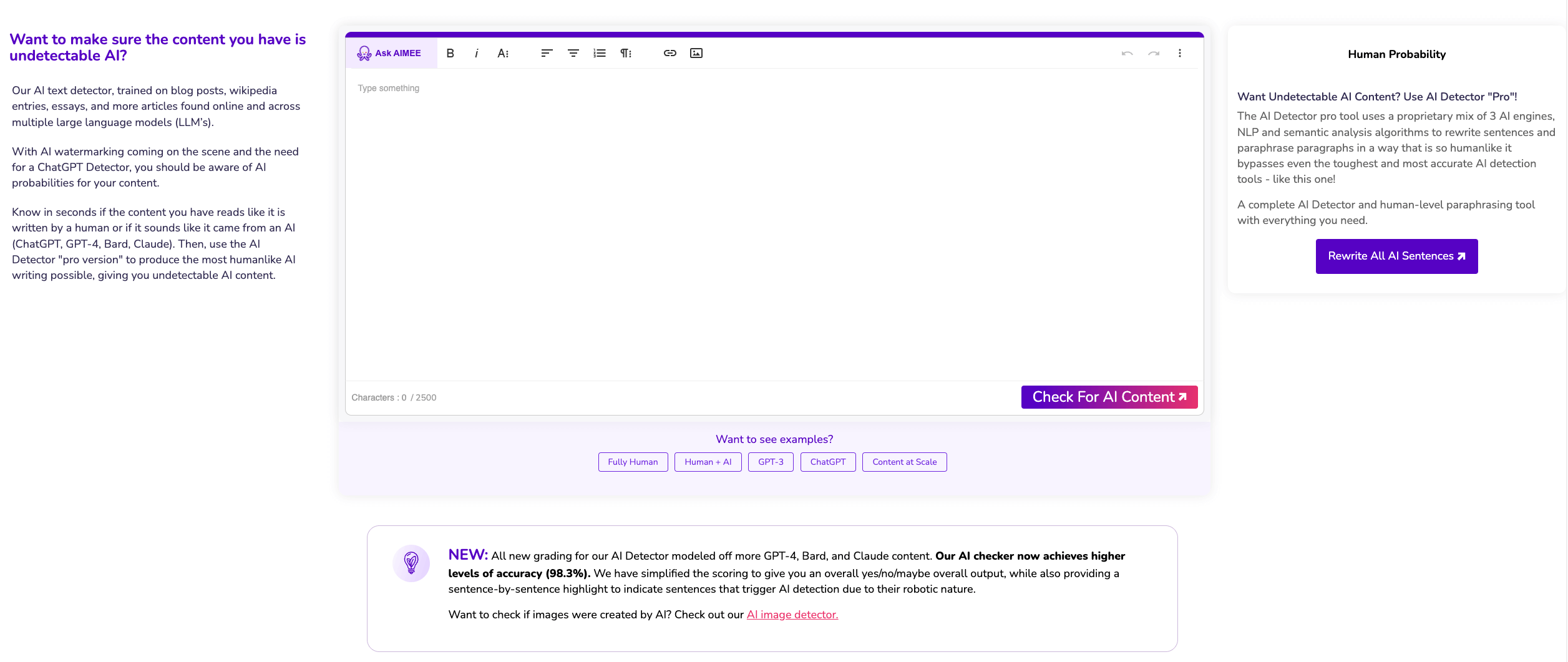The image features a horizontally rectangular layout set against a primarily white background. At the top left, bold purple text reads, "Want to make sure the content you have is undetectable AI." Beneath this heading, a smaller body of text explains the use of an AI test detector trained on various sources such as blog posts, Wikipedia entries, essays, and other articles found online and across multiple large language models.

To the right of this explanatory text, there is a horizontally aligned rectangular input box designated for text entry. Adjacent to it on the right side, a smaller informational box displays the phrase "Human Probability," paired with the call to action, "Want undetectable AI content? Use AI Detector Pro." This box is divided into sections, and at the bottom, against a purple background, features a prominent button labeled "Rewrite all AI sentences."